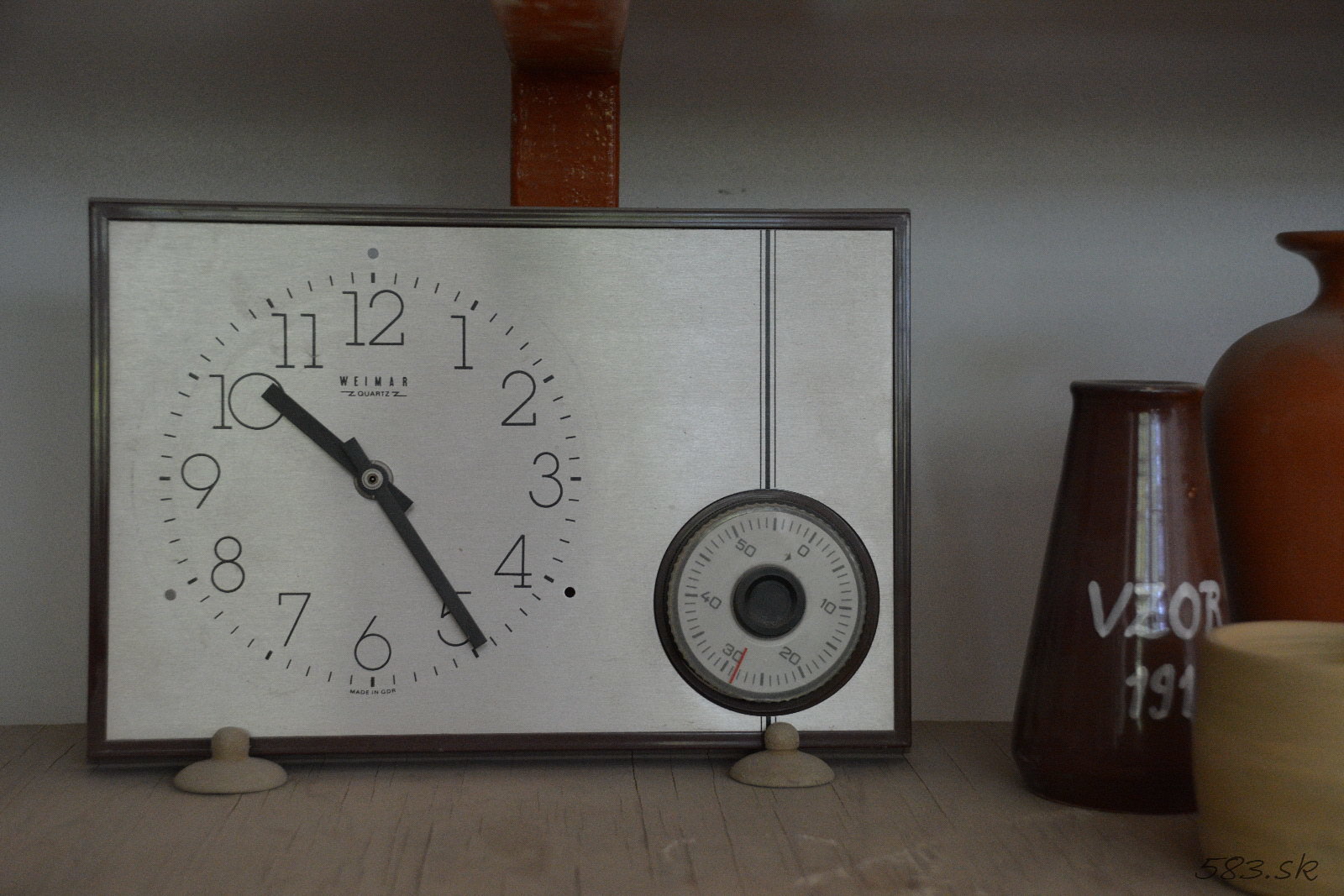The image displays a detailed scene of an analog clock leaning against a white wall with a light brown wooden floor below. The clock, encased within a rectangular picture frame supported by two wooden canisters, features thick black hour and minute hands pointing towards 10:25. Above the hands, the text "Weimar Courts" is inscribed. To the bottom left, a small analog timer marked in black, with a red hash mark near the 30-second mark, extends from a black cylindrical border that runs from top to bottom. On the right of the clock, three objects are arranged: a dark chocolate brown vase with white lettering "VZOR 191," an orangish-brown vase, and a beige wooden cup. The setting includes a white wall intersected by a reddish-brown beam, and in the image's lower right corner is the text "583.SK." The photograph is a close-up, highlighting the intricate features and color contrasts within the scene.